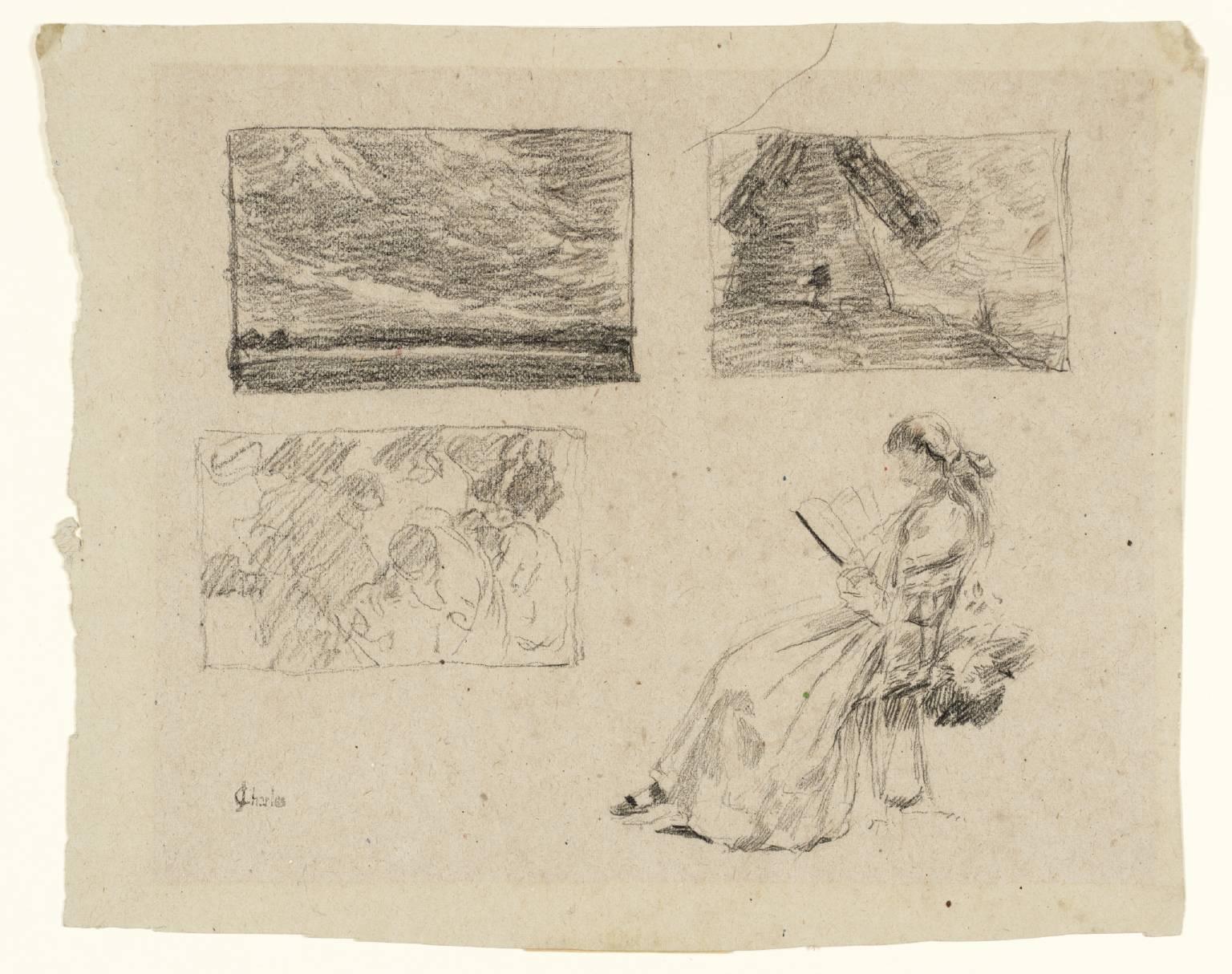This is an intricate series of pencil sketches on a worn, brown piece of paper with a square pink background, giving it an aged and artistic appearance. The paper features four distinct sketches arranged thoughtfully: 

In the upper left corner, there's a simple landscape sketch depicting the sky and land, possibly including a mountain. To the right of this, an old windmill or grain mill stands prominently, where a lone figure can be seen. Below these, on the lower left side, there's a more abstract sketch that appears to show a congregation of people. The most elaborate piece is in the lower right corner, illustrating a woman in Victorian-era clothing, sitting and slightly reclined, holding and gazing at an object in her hands, possibly a book. The lower left corner of the paper bears a signature, adding a personal touch to the compilation of these evocative images.